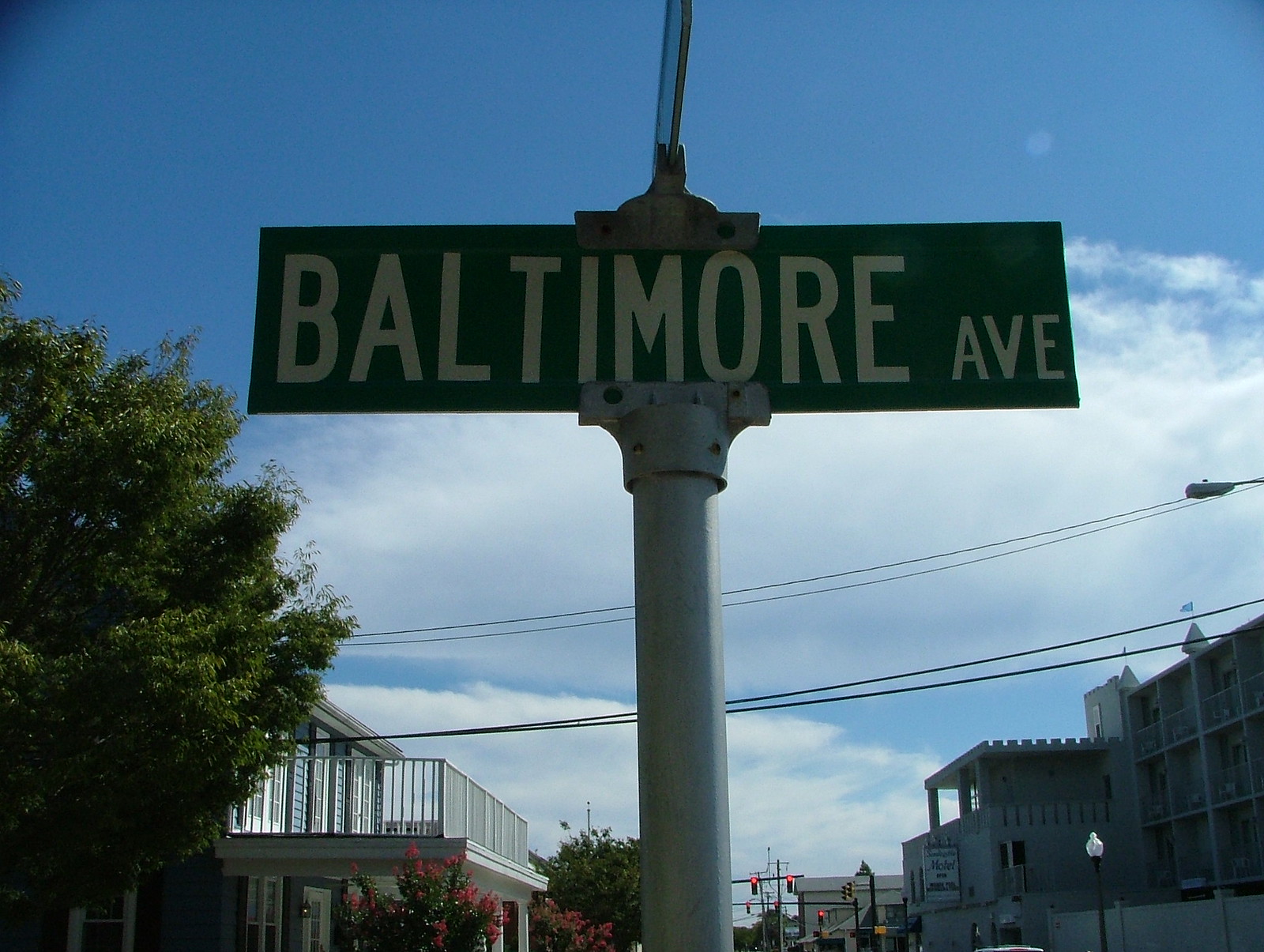In this detailed outdoor photograph, the central focal point is a prominent street sign displaying "BALTIMORE AVE" in bold, white capital letters. To the left of the sign, a lush green tree stands tall, providing a touch of nature. Adjacent to the tree, there is a building that appears to be a house, characterized by its large second-story porch adorned with white railings. The house itself is painted a subtle blue, adding a charming contrast to the scene. A bright blue sky with minimal cloud cover indicates a sunny day. A telephone wire stretches horizontally across the picture, adding an element of modern infrastructure. To the right, a streetlight stands tall, along with additional buildings that hint at a quaint urban neighborhood.